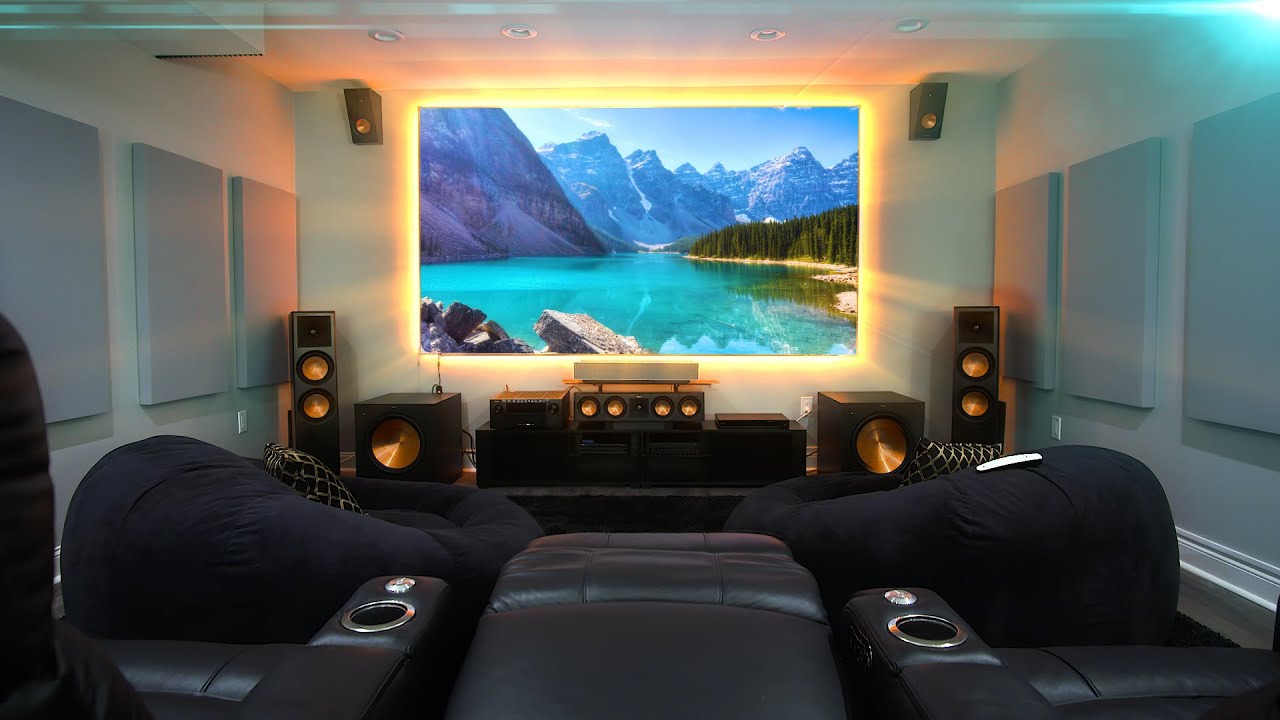The image depicts a sophisticated in-home studio designed for the ultimate movie-watching experience. The room features a trio of plush, black leather reclining chairs, complete with cup holders for added comfort, arranged at the back. In front of these chairs are two large, black bean bags, ensuring additional cozy seating options. The focal point of the room is an advanced entertainment system, which includes a substantial flat-screen TV showcasing an awe-inspiring, vibrant image of a mountain range and lake, with LED lighting providing a warm yellow back glow. Beneath the TV, the setup includes a state-of-the-art soundbar stereo system and various sleek black speakers arranged thoughtfully to enhance the surround sound experience. The room’s sleek, white walls create a striking contrast with the black furniture and entertainment equipment, imitating the ambiance of an authentic movie theater. Soundproofing padding on the side walls ensures an immersive, undisturbed audio experience, while a ceiling-mounted projector adds to the cinematic feel.